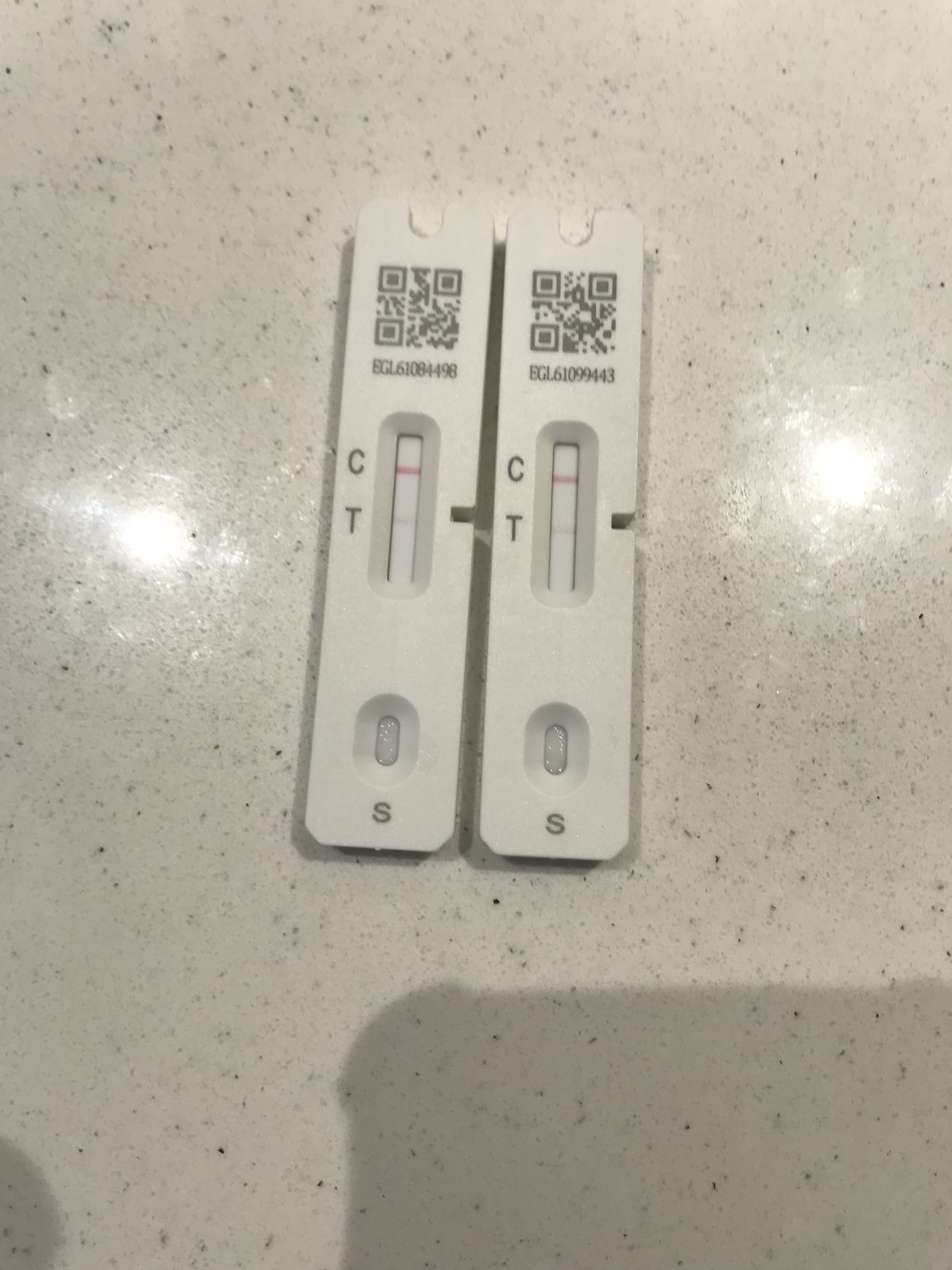The image features a marble-style background surface, upon which two identical COVID-19 rapid test kits are placed side by side. Each test is a small rectangular plastic device designed to indicate the presence of the virus using a saliva sample. At the top of the tests, there is a QR code that can be scanned for more information. Below the QR code, there is a test strip marked with the letters "C" and "T," where the results are displayed. Moving further down, there is a small well marked with an "S" for the placement of the saliva sample mixed with a solution.

In both tests, a strong red line appears next to the "C," which typically serves as a control line to indicate that the test has worked properly. Next to the "T," there is a faint line visible on both tests; however, the image does not clarify whether this faint line signifies a positive or negative result for COVID-19. The composition of the image is simple, including only the marble background and a shadow, likely cast by the phone used to take the photo.